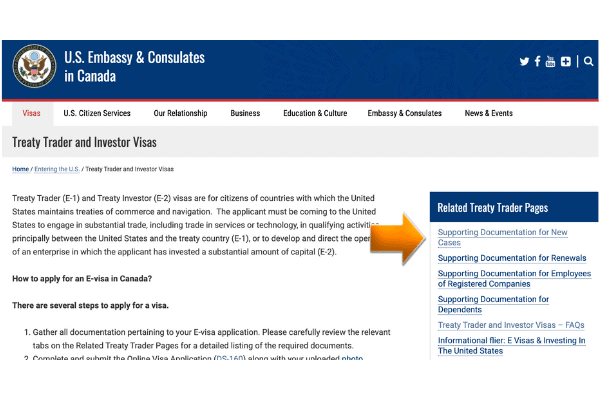This image is a screenshot from the U.S. Embassy and Consulates in Canada's website, specifically focusing on treaty trader and investor visas. The layout features black text on a white background, with a blue banner at the top. The webpage provides detailed information on how to apply for an investor visa in Canada, outlining key steps and necessary procedures. Highlighted by a yellow arrow, a menu page on the site lists various related topics including supporting documentation for new cases, renewals, employees of registered companies, dependents, treaty trader and investor visas, FAQs, an informational flyer, e-visas, and investing in the United States. The main text explains that treaty trader and investor visas are designated for citizens of countries with which the United States has treaties of commerce and navigation. It specifies that applicants must be traveling to the U.S. to engage in substantial trade, including services or technology, in qualifying activities primarily between the U.S. and the treaty country, or to develop and direct an enterprise where they have invested significant capital.